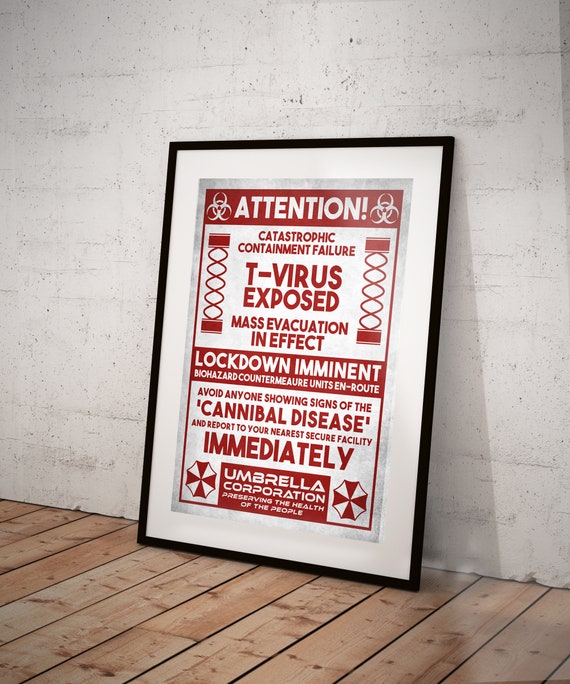The image depicts a framed poster leaning against a whitewashed brick wall with a highly polished, light wood plank floor. The frame of the poster is black with a white matting that accentuates the vivid red and white poster inside. At the top, in large white letters against a red background, the poster reads "Attention!" followed by an exclamation point. The text on the poster warns of a "Catastrophic Containment Failure" and states that the "T-virus" has been exposed, necessitating a "Mass Evacuation in Effect." Further, it indicates that a "Lockdown" is imminent and "Biohazard Countermeasure Units" are en route. The poster advises avoiding anyone showing signs of a "cannibal disease" and instructs individuals to report to the nearest secure facility immediately. At the bottom, it identifies the "Umbrella Corporation," noting their motto: "Preserving the health of the people." The poster also features biohazard symbols and decorative designs along the sides, resembling a vintage or movie prop warning sign.